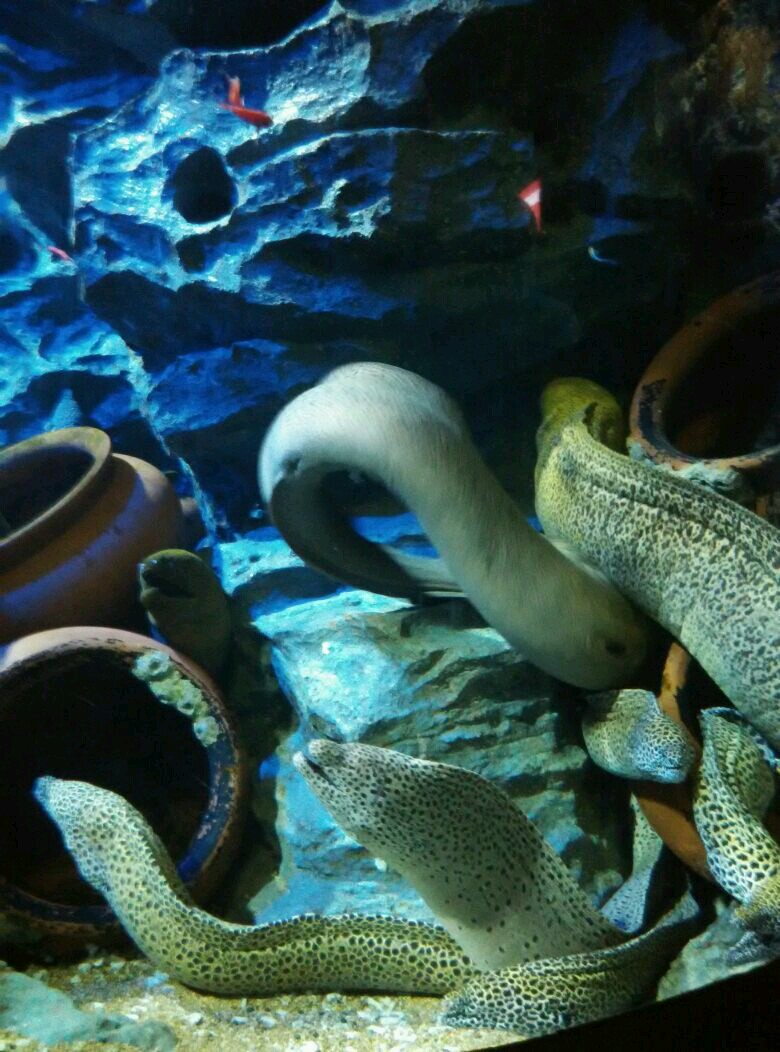This photograph captures an elaborate underwater display, likely within an aquarium. The scene features several sea eels with varied appearances—some are white with black spots, others are solid white, and a few exhibit a light green color speckled with dark spots. These eels are actively swimming, intertwining with one another, and gliding in and out of the broken terracotta pots scattered on the white sandy bottom. The backdrop is composed of blue-tinged rocks, suffused with blue light, adding a surreal ambiance to the scene. Notably, there are hints of reddish hues on the rocks, possibly from other sea creatures or decorative elements. This detailed and dynamic underwater environment effectively showcases the eels as they navigate the intricate arrangement of terracotta pots, sand, and illuminated rocks.